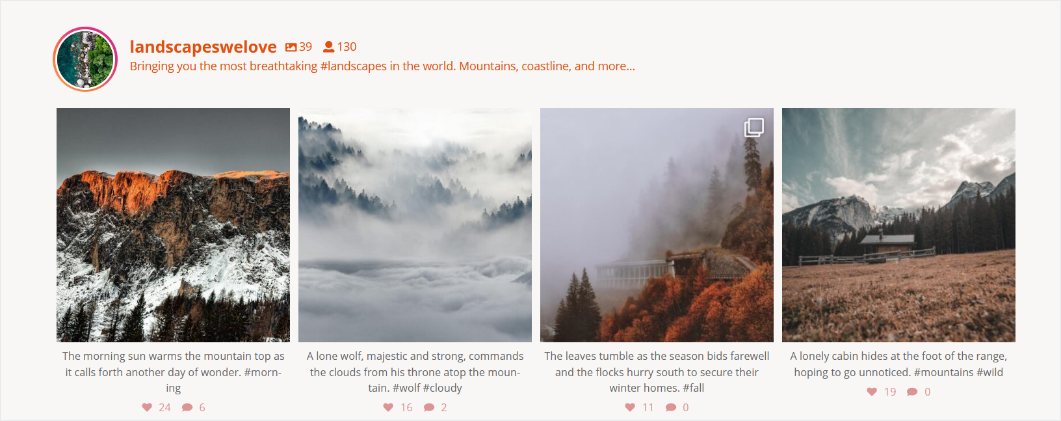This screenshot, displayed in landscape mode, features a structured, two-section layout set against a subtly darkened white background. 

**Upper Section:**
- **Avatar:** A circular icon in shades of pink and orange. Within the circle, a lush green forest with a silver line down the middle can be partially seen.
- **Text Labels:**
   - **Title:** "Landscapes We Love" in orange.
   - **Statistics:** "39 images" and "130 members."
   - **Tagline:** "Bringing you the most breathtaking #landscapes in the world. Mountains, coastlines, and more."

**Lower Section:** 
- **Subdivided into two subsections.**
  - **Left Subsection:** Features four images, each with corresponding descriptions.
    1. **First Image:** A snowy mountaintop. Underneath, it reads: "The morning sun warms the mountaintop as it calls forth another day of wonder. #morning." This image has garnered 24 likes and 6 comments.
    2. **Second Image:** Described as a lone wolf atop a mountain, commanding the clouds. Accompanied by hashtags: #wolf, #cloudy. However, the wolf is not visible in the image.
    3. **Third Image:** Depicts autumn leaves tumbling, with a description mentioning the seasonal change and flocks of birds migrating. The birds are not visible.
    4. **Fourth Image:** Shows a lonely cabin nestled at the foot of a mountain range, with the caption: "A lonely cabin at the foot of the range, hoping to go unnoticed." This image is noted for its beauty.